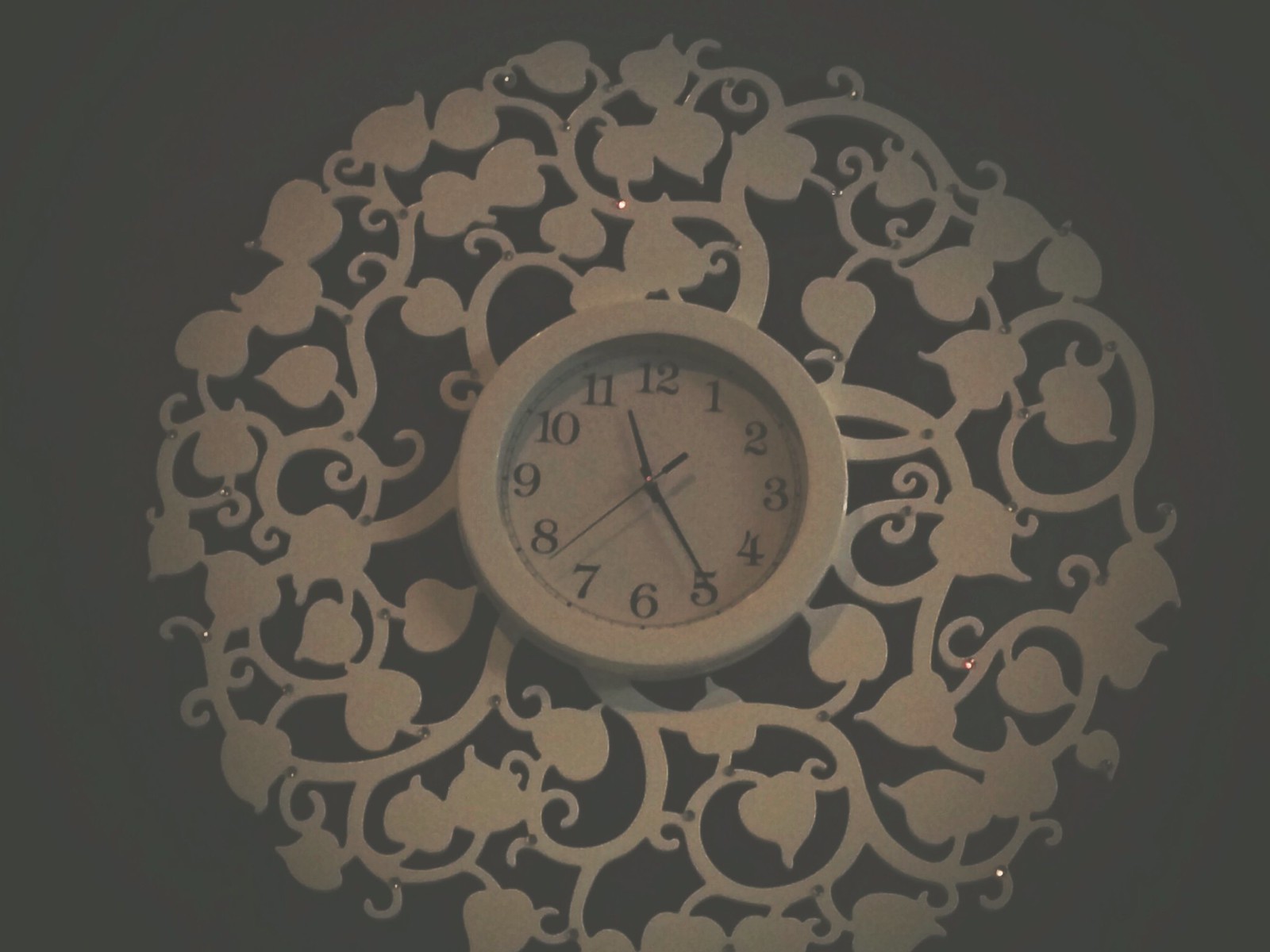This image showcases a wall-mounted clock with a distinctive and elaborate frame. The clock itself has a classic design with a white face, black numerals, and matching black hour, minute, and second hands. The standout feature of this clock is its oversized, ornate frame, which adds a touch of elegance and sophistication to an otherwise basic timepiece. The frame is intricately decorated with floral patterns that appear to be finely detailed, giving the impression of a metal craftsmanship, although it is likely made from plastic. The frame is securely attached to the wall with several visible bolts, ensuring stability. This decorative frame significantly enhances the visual appeal of the clock, making it a striking centerpiece on the wall.